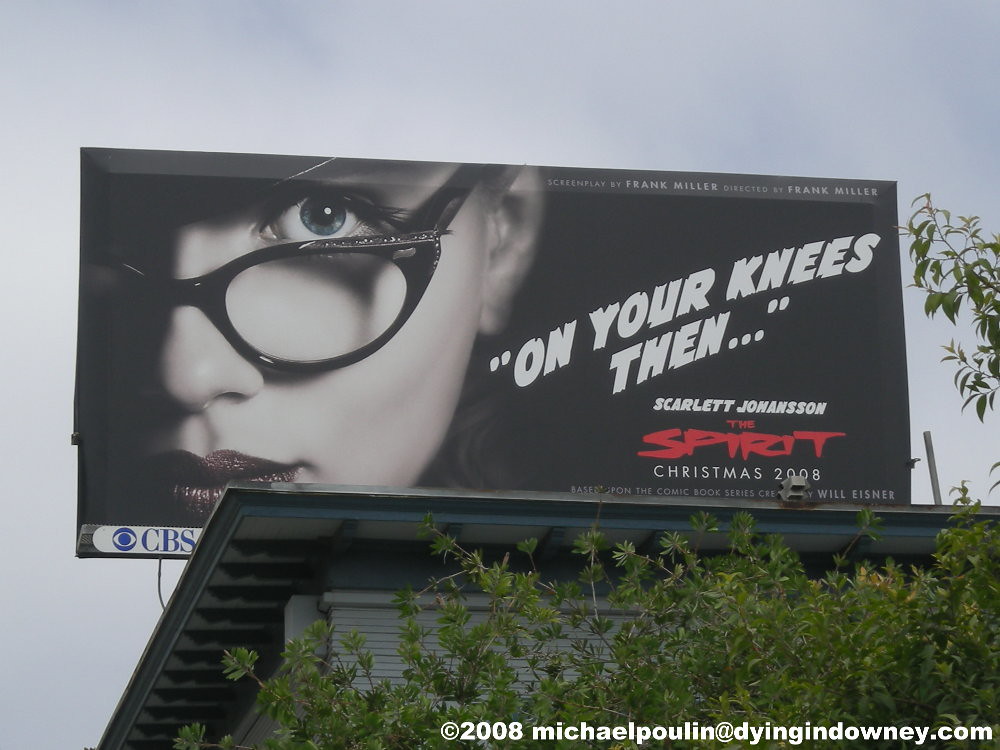Title: Billboard for CBS Television Show "The Spirit" Featuring Scarlett Johansson

Caption: This striking billboard advertisement for the CBS television show "The Spirit," set to premiere during Christmas of 2008, commands attention with its dramatic design. The large billboard is perched atop a building and features a predominantly black background. Dominating the left side is a half-cut off, black-and-white image of a Caucasian woman's face, identified as Scarlett Johansson. She dons vintage, black plastic-rimmed glasses circa the 1960s, characterized by their slight winged corners. Only one eye is visible, though its color remains indiscernible due to the monochromatic scheme. Her lips are painted, but the exact shade of her lipstick is also unclear.

Overlaying the image, the text “on your knees…” appears in white, strikingly placed to add an element of intrigue. Below, Johansson's name is prominently displayed, with "Scarlett Johansson" appearing in both white and red lettering. The show's title, "The Spirit," is written in larger, stylish letters, with the words "Christmas of 2008" indicating the premiere date beneath it.

In the bottom right corner, the text "© 2008 Michael Poulin at Dinedowney.com" serves as a copyright note, crediting the photographer and his website. This visually arresting billboard not only highlights the star power of Scarlett Johansson but also teases the mysterious and captivating nature of the upcoming show.